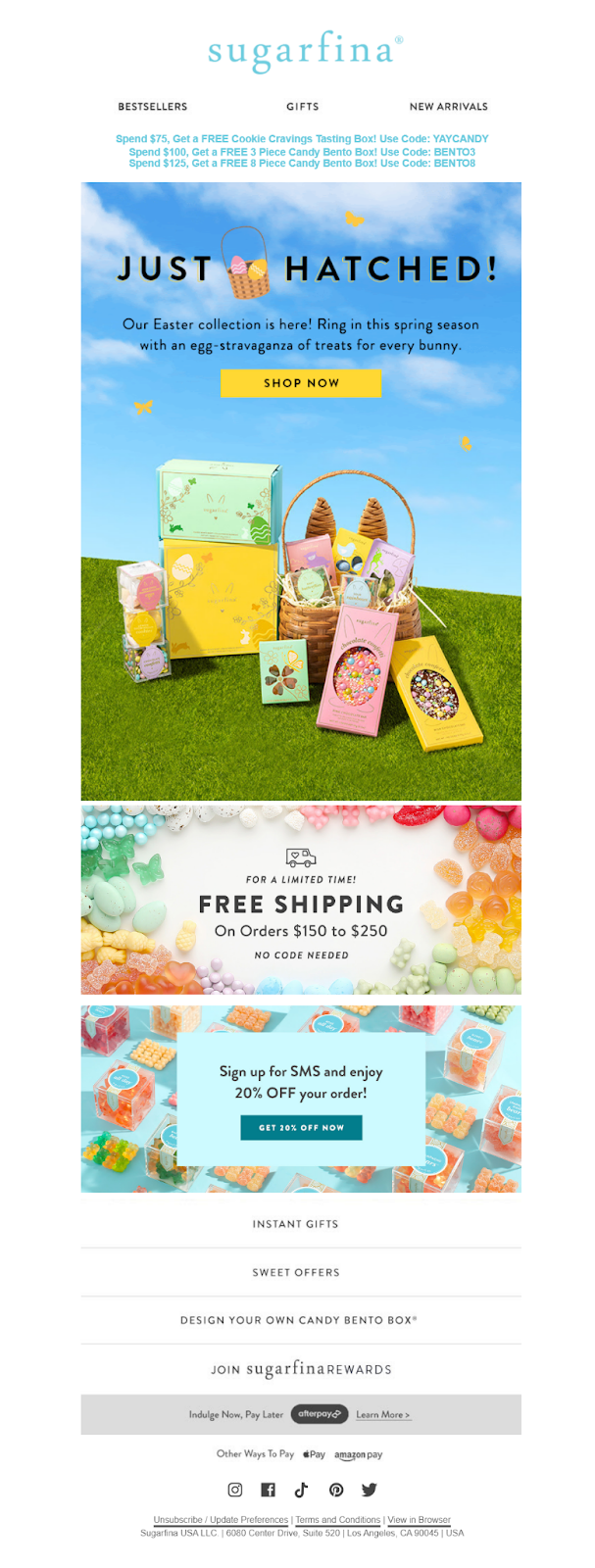Here is a detailed and cleaned-up caption for the image:

---

The image displays a lengthy website layout that appears to originate from an email. At the top center, there is the "Sugarfina" logo. Below the logo, there are three navigation buttons labeled "Bestsellers," "Gifts," and "New Arrivals." Further down, promotional offers are presented: 

- Spend $75 and receive a free Cookie Cravings Tasting Box with code "YAYCANDY."
- Spend $100 and get a free three-piece Candy Bento Box with code "BENTO3."
- Spend $125 and obtain a free five-piece Candy Bento Box with code "BENTO5."

The next section highlights a seasonal promotion with the banner "Just Hatched! Our Easter Collection is Here." The description urges customers to "Ring in the Spring Season with an Egg-stravaganza of Treats for Every Bunny," and features a prominent yellow "Shop Now" button.

Following this, another promotional offer is displayed, stating, "For a limited time, free shipping on orders $150 to $250. No code needed."

At the bottom of the image, a section promotes signing up for SMS alerts with the promise of a 20% discount on the next order. This section also mentions benefits like "Instant Gifts," "Sweet Offers," the ability to "Design Your Own Candy Bento Box," and an invitation to "Join Sugarfina Rewards."

---